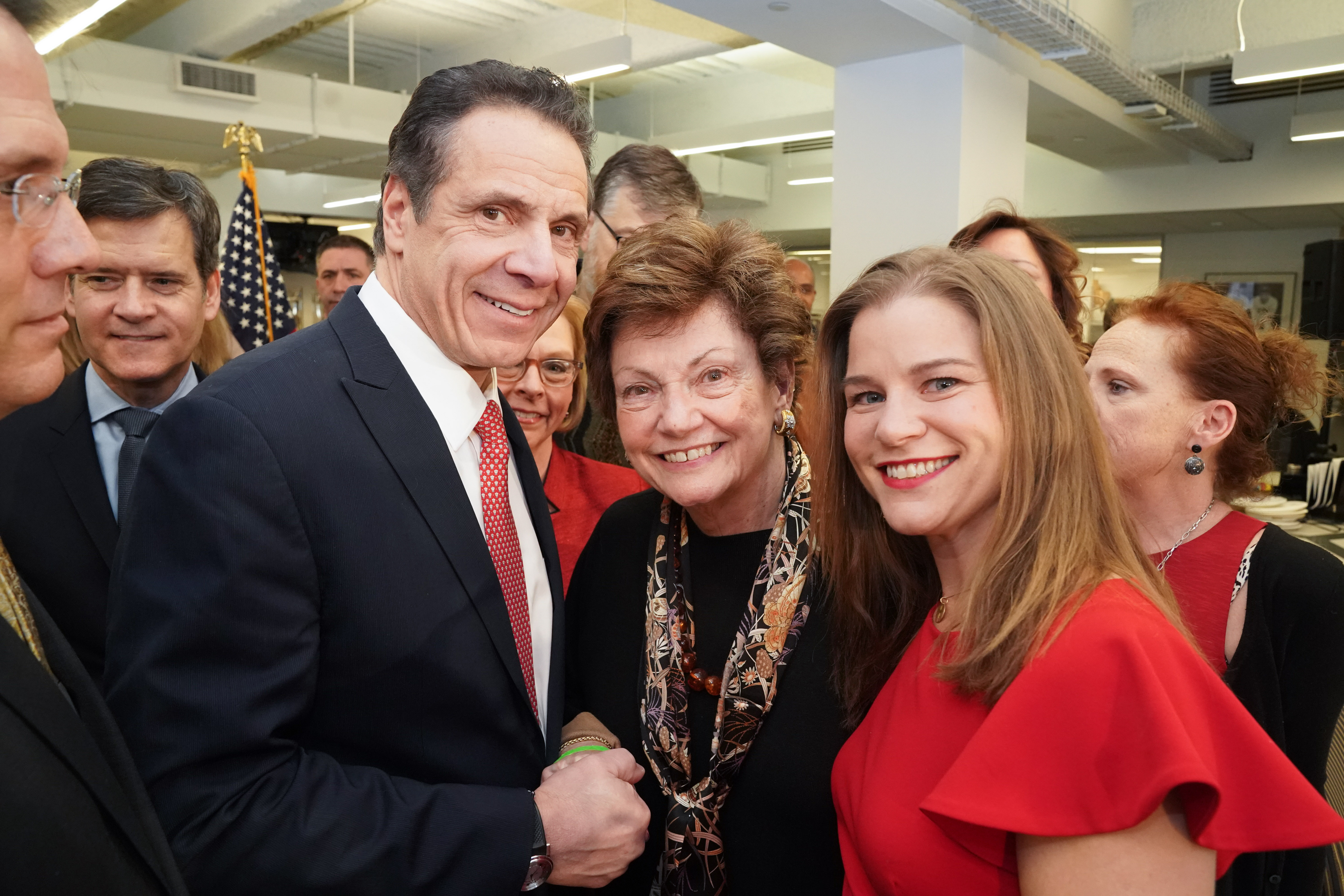This photograph captures a group of people at a political event inside an office setting, with three individuals as the primary focus. On the left stands a white male, likely in his 50s, with medium-length dark hair combed back. He is dressed in a black suit, white shirt, and a red tie adorned with white dots, giving the impression of being a politician. He is shaking hands with a white female to his right, who appears to be in her 60s. She has short brown hair and is adorned with large gold hoop earrings, a black, white, and gold floral silk scarf around her neck, and a brown beaded necklace over her black top. To her right stands a younger white female, possibly in her 20s or 30s, with shoulder-length brown hair and blue eyes. She is smiling and wearing a red blouse. Behind them, several people dressed in business attire are watching and smiling, enhancing the formal and professional atmosphere. American flags can be seen in the background, and the setting is adorned with doorways, walls, and some artwork, indicating an indoor office environment.